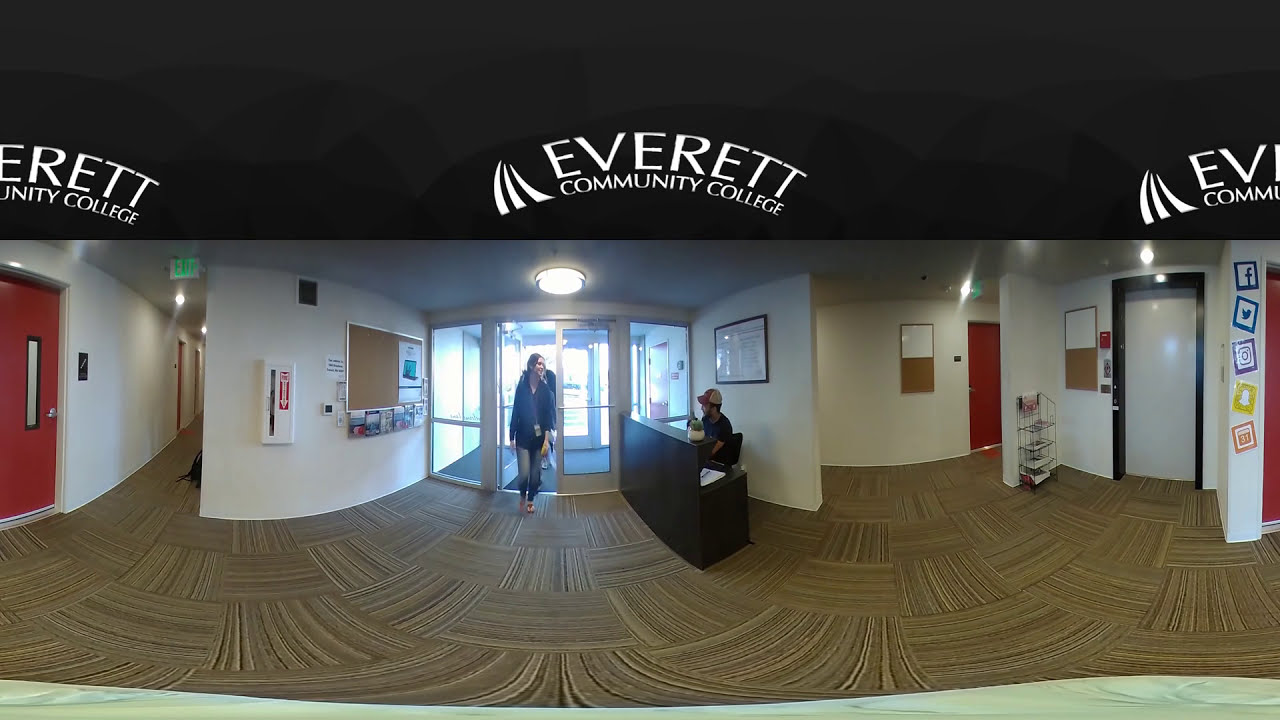In the center of the image is the entrance to Everett Community College, marked by a sign above the automatic sliding glass doors. A young woman is entering through these doors, while to her right, a man in a red trucker hat is seated behind a brown wooden receptionist desk. The receptionist is greeting the woman. Behind him is a partition wall with a framed directory.

The walls on the left side of the entrance are white and feature a cork board with several flyers and a fire extinguisher within an emergency casing. Adjacent to this wall is a hallway with a green exit sign on the ceiling and a red door at the very left end. Inside the lobby area, the floor is carpeted with a pattern of different lines, creating a distinct ambiance.

The walls on the right side of the entrance display various social media logos, including Facebook, Twitter, Instagram, and Snapchat. Additionally, a bulletin board is visible on this side. Further into the room, past the reception desk, is another door, possibly leading to a classroom. This detailed scene provides a comprehensive view of the college's welcoming entrance, combining elements like the reception area, informative displays, and clear signage.